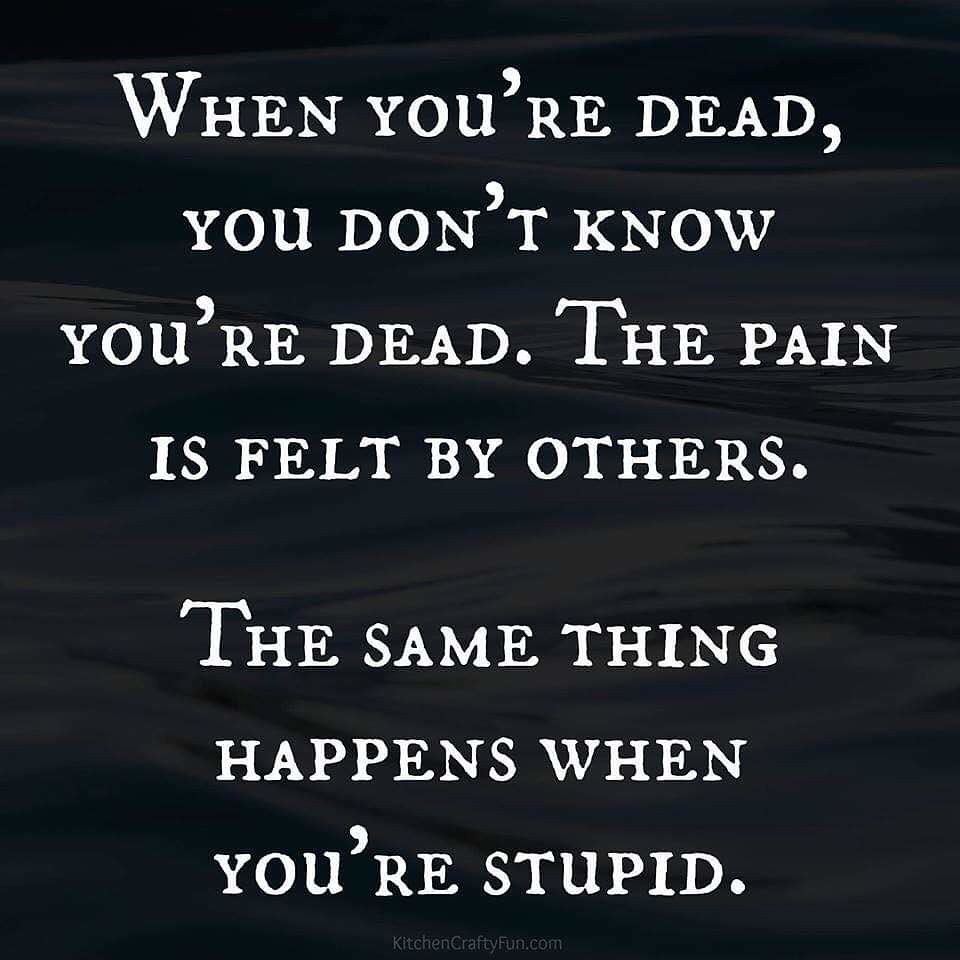The image features a quote displayed in white text on a black background that has a textured appearance, resembling either water waves or wood grain. The text reads: "When you're dead, you don't know you're dead. The pain is felt by others. The same thing happens when you're stupid." The quote is presented in two distinct paragraphs, adding emphasis to the punchline. At the bottom of the image, the source is noted as "KitchenCraftyFun.com," with capitalized letters for each word. The overall aesthetic, with its striking simplicity and textured backdrop, lends the quote a Twilight Zone-like feel. The oversized commas and plain font style give it a familiar, internet meme quality, making it easily shareable and likely to resonate on social media platforms.